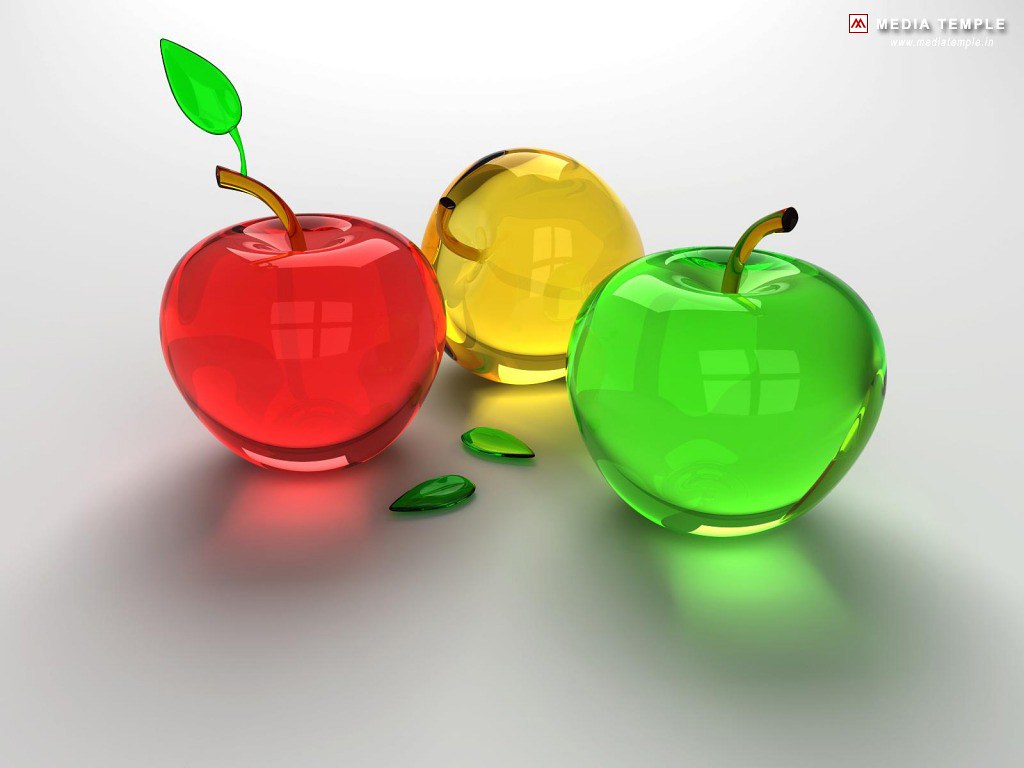This image features three vibrant glass apples displayed on a shiny white surface, set against an off-white to gray background. The apples are positioned centrally, with the red apple to the left, the yellow apple in the middle, and the green apple to the right. The red apple, standing upright, showcases a bright green glass leaf attached to its brown stem. In contrast, the yellow apple lies on its side with its brown stem pointing upwards, while the green apple stands upright, its brown stem tilting slightly to the right. On the white surface, between the apples, rest two fallen green glass leaves. The top-right corner of the image is marked with the small white text "Media Temple," accompanied by a red box containing an "M." The vivid glass apples and their delicate glass components cast subtle shadows, adding to the image's intricate detail.